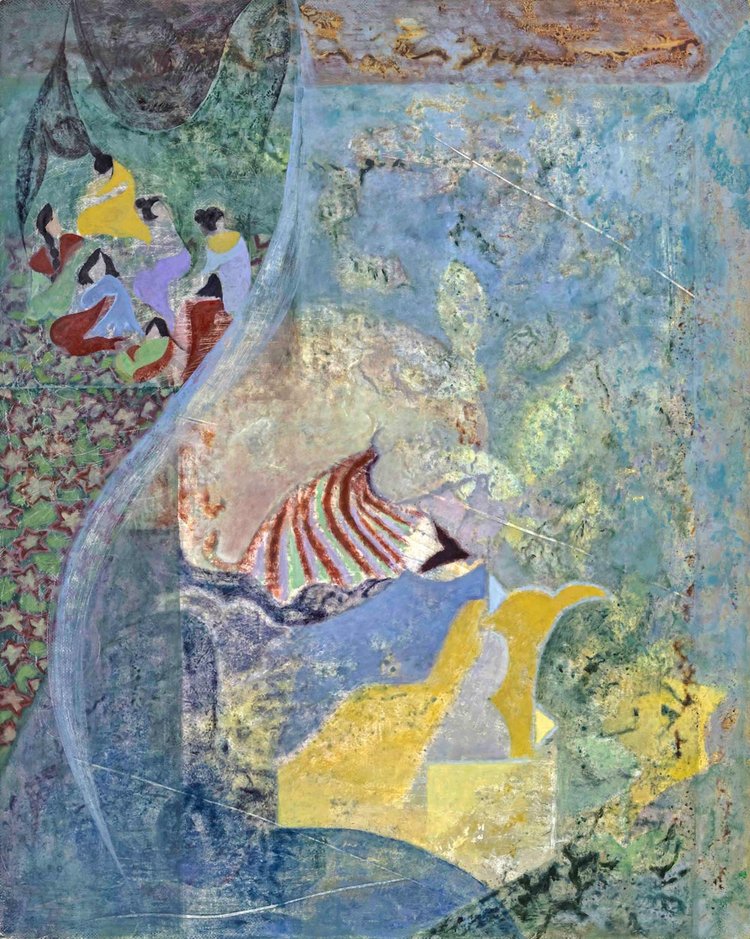This painting, displayed on an earthy, rocky surface in some disrepair, exhibits an abstract and impressionist style incorporating a range of colors and motifs. The upper left portion of the artwork features groups of seven young women with black hair, clad in robes of blue, yellow, purple, and light blue. They appear to be looking towards the upper right of the image, set against a greenish background adorned with faint red-outlined stars. The lower section transitions from a predominantly blue area into assorted yellow shapes, including forms akin to a square, a banana, and a triangle, intricately positioned. Towards the deep center, there exists a swirling pattern of red, green, and white hues. On the upper right side, a faded orange block contrasts sharply with the overall light blue background. Additionally, the blue area to the right highlights faint, possibly aquatic designs like outlines of fish and a partly visible seashell, characterized by red stripes and a green backdrop. The entire mural demonstrates a striking yet weathered blend of colors and abstract figures that create a captivating visual narrative.